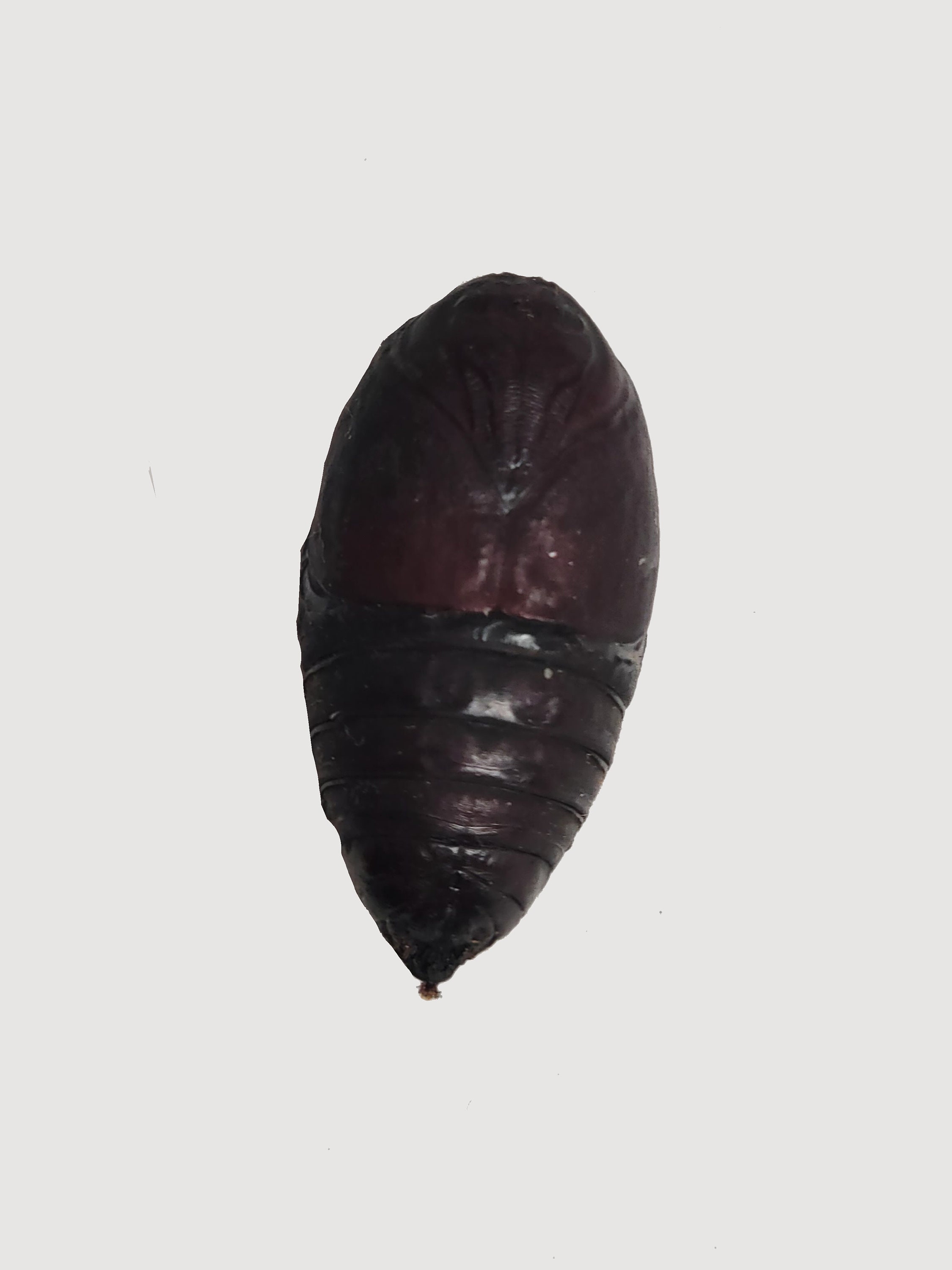The image features a striking, almond-shaped object with a soft gray background, creating a simple yet captivating focal point. The object is round at the base, positioned at the top of the picture, and tapers to a pointed end at the bottom. The upper half of the object is a softer, lighter bronze or dark brown tone, while the lower half transitions into a darker bronze or near-black color. Distinctive horizontal ridges run across the entire object, giving it an intricate texture. This makes it resemble natural elements like a seed, bean, or perhaps even an insect pupa or fossil. The object has an oblong shape with a pointy tip at the bottom, where a small, tassel-like extension can be observed. Despite its ambiguous nature, the object's detailed coloring, shape, and texture invite various interpretations, ranging from botanical to entomological elements.